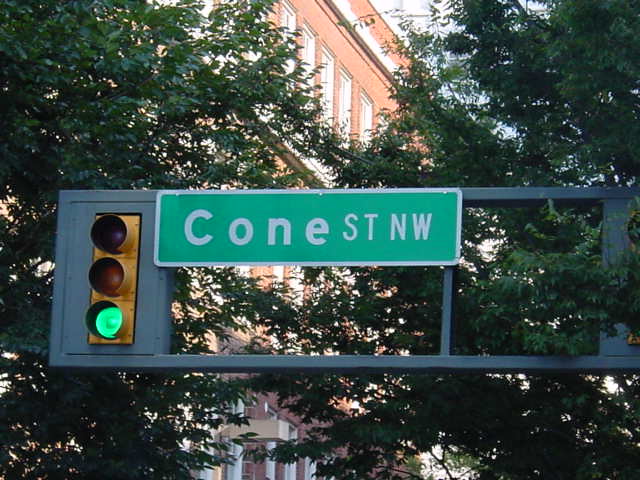A close-up photograph captures a street sign and traffic light embedded into a metallic overhang, hanging over the street. The traffic light signals green. The rectangular metal base supports a street sign that reads "Cone Street Northwest" in bold white letters on a light green background. In the upper part of the image, a very large red brick building with numerous windows dominates the background. The scene is framed by two lush, green trees on either side, whose branches intersect, giving the impression of a single, expansive tree. Steel lines run from the right side of the image to support the traffic light holder on the far left. The image, taken outdoors, showcases the urban setting with the tall building, which could resemble an office or hospital, beyond the greenery. We do not see the road or any vehicles below, only the streetlight and the surrounding elements.